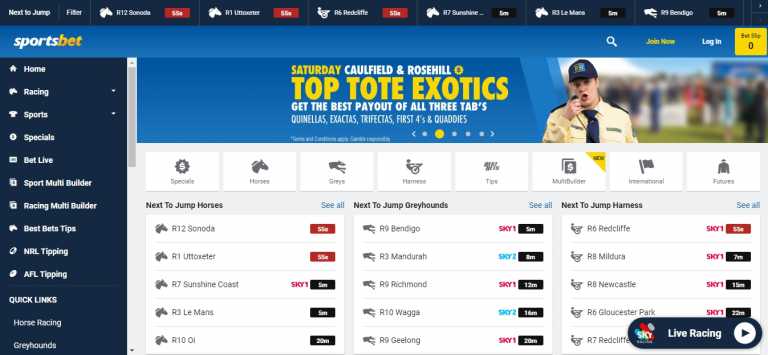The image displays a slightly blurry webpage dedicated to horse racing betting, making some details difficult to read. The top section of the website features a navy blue banner with a heading that reads "Next to Jump" and "Filter," accompanied by a graphic of a horse. Below this heading, there are numerous horse names, each paired with a red box indicating the option to place a bet. Adjacent to this, the banner includes a row labeled "Sports Bet," where "BET" is highlighted in yellow while "Sports" is in white.

On the left-hand side of the webpage, a vertical column lists various categories, each represented by an icon with corresponding text to its right. This includes a home icon for "Home," a horse icon for "Racing" with a dropdown menu, a jersey icon for "Sports" with another dropdown menu, and possibly a clock icon for "Specials." Other options in the column include "Bet Live," "Sport Multibuilder," "Racing Multibuilder," "Best Bet Tips," "NRL Tipping," "AFL Tipping," "Quick Links," "Horse Racing," and "Greyhounds."

Towards the right side of the page, a broad banner in blue extends over three separate columns. It is titled "Saturday Caulfield and Rose Hill Top Tote Exotics. Get the best payouts of all three tabs." Below this banner lies a row containing various categories like "Specials" and "Horses." Further down, the webpage is divided into three key sections: "Necks to Jump Horses," "Necks to Jump Greyhounds," and "Necks to Jump Harnesses," each listing multiple names and options to bet on.